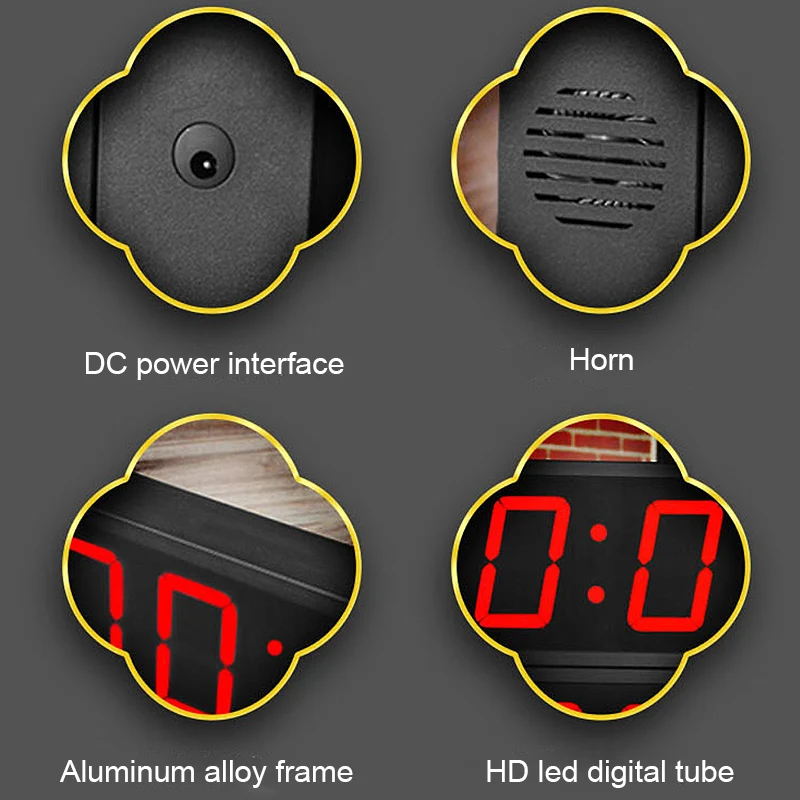This image, potentially an advertisement or a part of a textbook, features a detailed display of components against a gray background, possibly relating to an alarm clock or electronic device. The layout comprises four distinctly outlined sections, each highlighted with a yellow or gold border. 

Starting from the top-left, the first section showcases a black "DC power interface," indicating the spot where power is plugged into the device. Next to it, an image labeled "horn" displays what seems to be a grate on the side, likely for sound emission, and is marked with the same yellow or gold outline.

The bottom-left section focuses on an "aluminum alloy frame," illustrated as the structural frame of a digital clock. Finally, the bottom-right section highlights an "HD LED digital tube," emphasizing the area where the clock's digital numbers are displayed, with visible red digits "0" and "0."

Overall, this image appears to be a comprehensive display board, effectively illustrating key parts of a digital clock or similar electronic product for educational or advertising purposes.